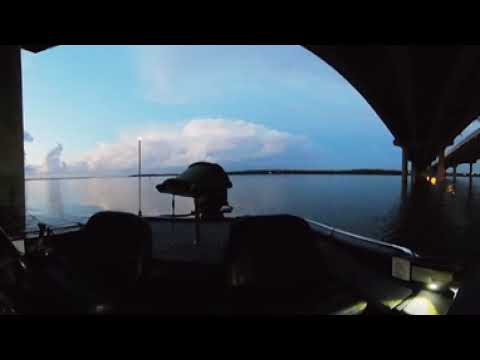In this photograph, we see a boat or raft positioned under an elevated, multi-lane bridge supported by massive pillars. The scene is predominantly dark due to the shadow cast by the bridge, creating deep contrasts. The boat, partially illuminated by a small light on the lower right, reveals minimal details; though an engine and possible seating are discernible, the specifics remain obscure. The water around the boat is calm, presenting a deep blue hue that contrasts with the dark shadows. To the right, additional pillars submerge into the water, further emphasizing the bridge's structure. In the background, a serene sky stretches with a large, white cloud at its center, adding a sense of tranquility to the scene. This juxtaposition of the dark, shadowy foreground and the bright, calm background creates a stark yet harmonious visual. The primary colors in the image are black, blue, white, along with touches of yellow and red, contributing to the overall serene and contemplative mood.